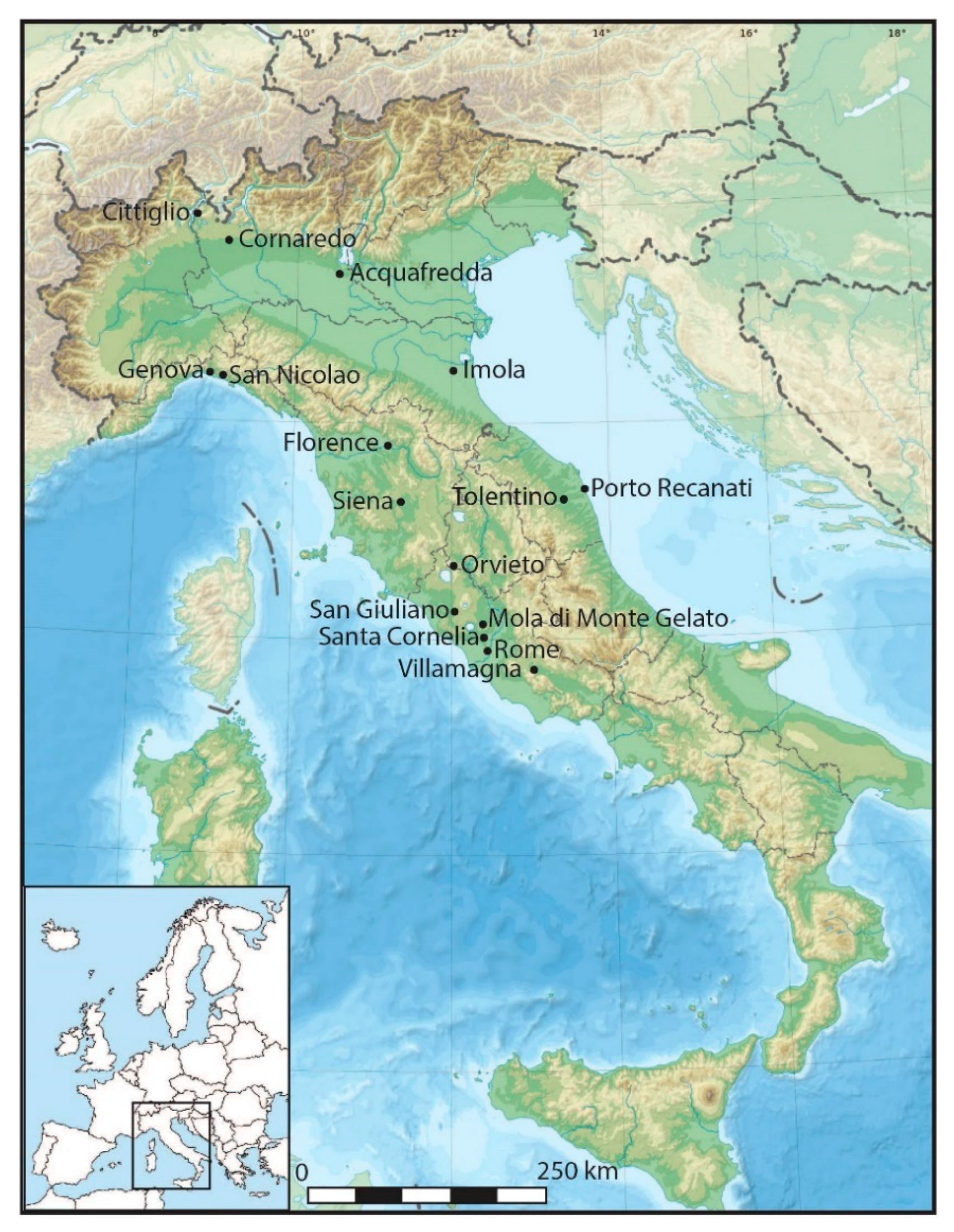The image is a detailed topographical map of Italy, showcasing the country's varied elevations with gradients from light green in the lowlands to darker greens and light tans at higher elevations, signifying the mountainous regions. Italy is surrounded by light blue waters, with bordering countries delineated in tan but left unlabeled. Prominently featured cities across Italy are marked with black dots and names in black font, including both well-known and lesser-known locations. Notable cities labeled on the map span from the north to the south, such as Florence, Siena, Genova, Imola, San Nicolao, Rome, and Villa Magna, as well as smaller locales like Cittiglio and Acquafredda. In the bottom left corner, an inset depicts a simplified map of Europe, highlighting Italy within a boxed area. This inset map presents Europe in white with black country borders. Additionally, there is a key indicating the scale of the map, illustrating that one inch represents 250 kilometers.